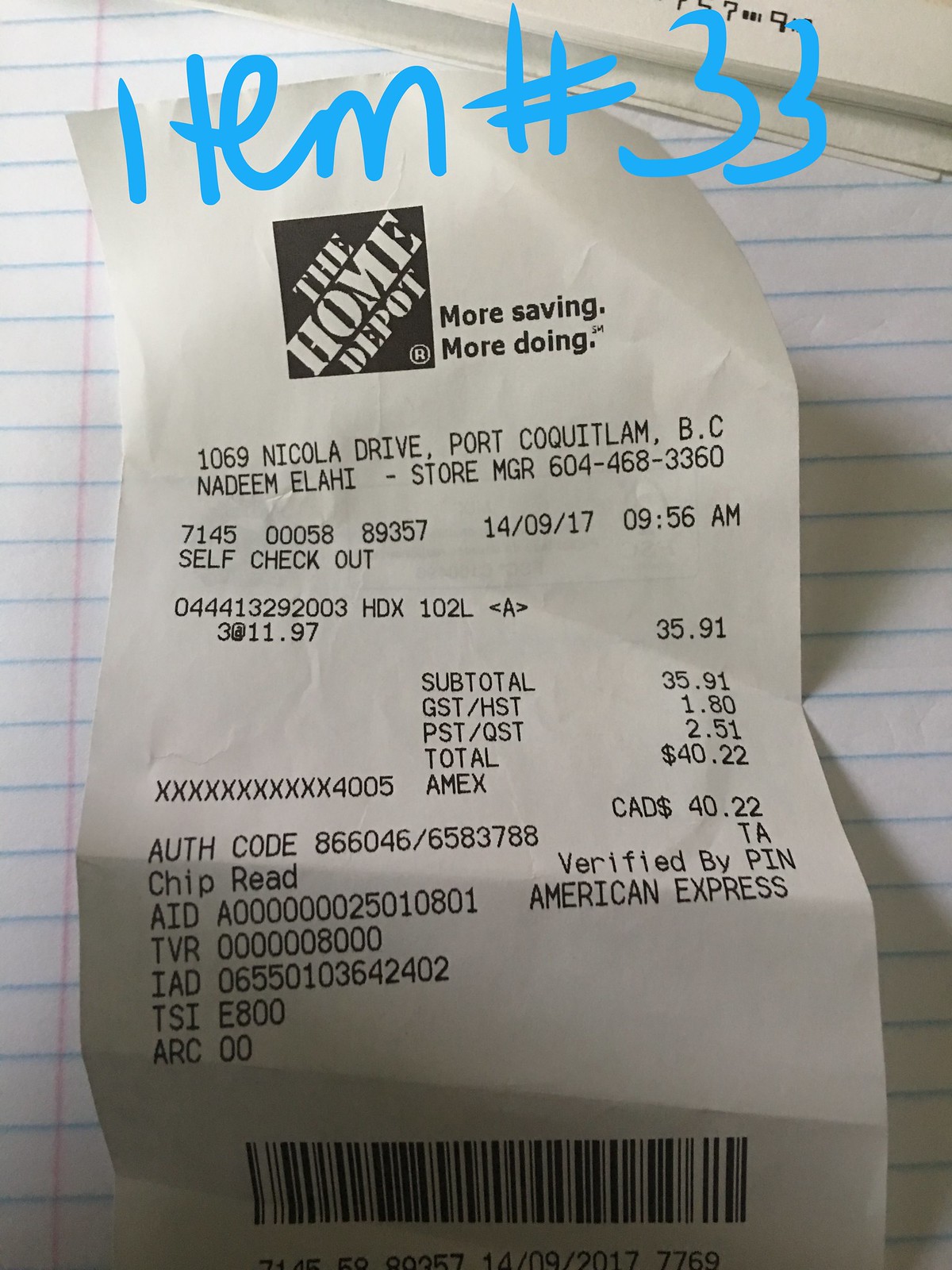This detailed close-up photograph captures a Home Depot receipt laid on top of a lined notebook paper. The receipt is slightly crumpled and occupies almost the entire frame, appearing to be from a Home Depot store located at 1069 Nicola Drive, Port Quantillam, BC, British Columbia, Canada. The top of the receipt displays the distinctive Home Depot logo—a black square with diagonal white text reading "The Home Depot®" and their slogan "More Savings. More Doing." Below this, the receipt provides various transaction details: it is managed by Nadeem Elahi (Store Manager), and showcases a purchase totaling CAD $40.22 paid via an American Express card, with a partial card number ending in 4005. Sales details include GST/HST of $1.80 and PST/QST of $2.51. The transaction details show a purchase at 09:56 AM at a self-checkout. Additional codes include an authorization code 866046/6583788 and various technical data elements like TVR, IAD, and TSI. At the bottom of the receipt, there's a barcode consisting of compact white and black lines. Overlaid on the image, written in blue hand-drawn text, is "item #33," suggesting it might be part of a collection or catalog. In the background, the lined notebook paper features dark blue horizontal lines and a singular pink vertical line. In the upper right of the image, other papers are partially visible, adding further context to the scene.